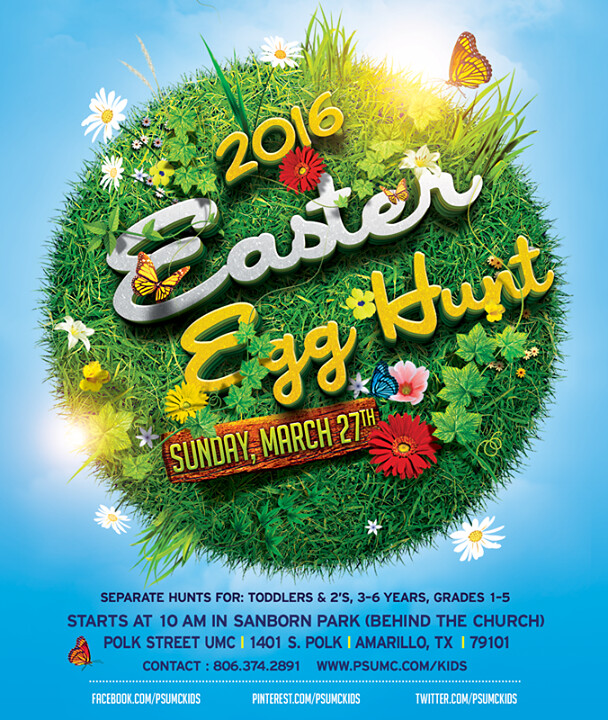The image is a detailed advertisement poster for a "2016 Easter Egg Hunt" event. The central focus is an artist's rendition of a round patch of grassy field adorned with daisies, various colorful flowers, and butterflies in hues of yellow, red, and blue. Amidst this vibrant scene, the prominent text "2016 Easter Egg Hunt" is displayed, along with the event date "Sunday, March 27th." Below the circular grassy artwork, the poster details that there will be separate hunts for different age groups: toddlers and two-year-olds, children aged three to six years, and kids in grades 1 to 5. The event starts at 10 a.m. and will be held at Sanborn Park, behind the church, Polk Street UMC, located at 1401 South Polk, Amarillo, Texas, 79101. Additionally, the poster provides contact information: phone number 806-374-2891, and a website www.sumc.com/kids. The background of the poster is a pale blue, and the text below the graphic is in black.